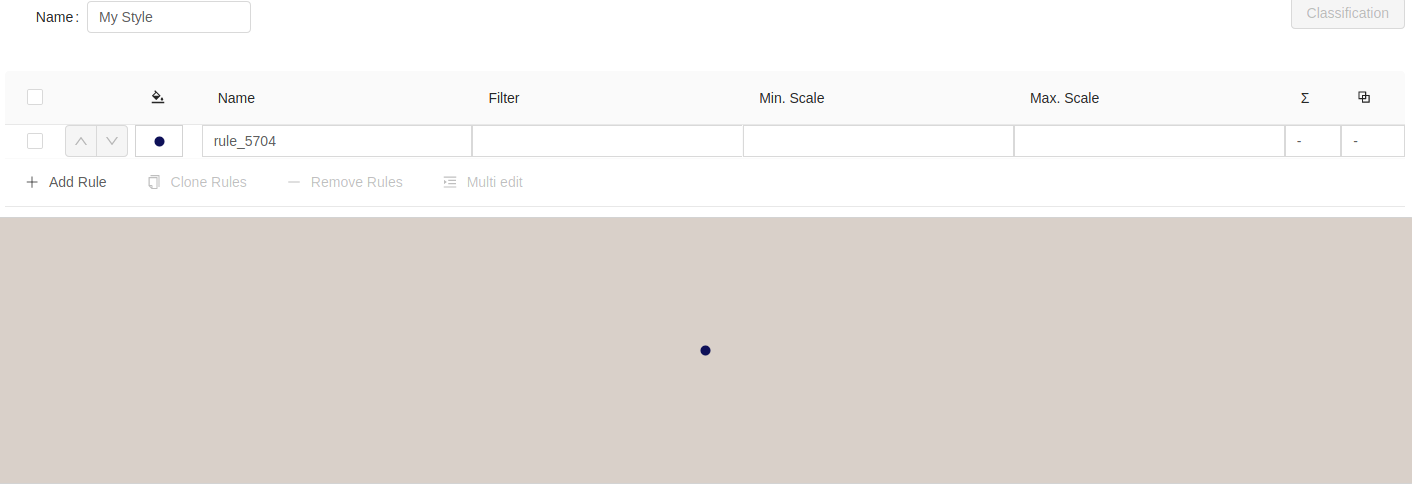The image appears to be a screenshot of a section of an online form on a website. At the top left of the form, there is a label that says "Name" with a corresponding small text box to the right that contains the text "My Style." Below this, there are several fields arranged in a vertical format. The first field also labeled "Name," has a text box beneath it with the entry "RULC_5704." Following this, there are fields labeled "Filter," "Min Scale," and "Max Scale." The lower half or remaining part of the screen is dominated by a large beige box with a single small black dot in the center.